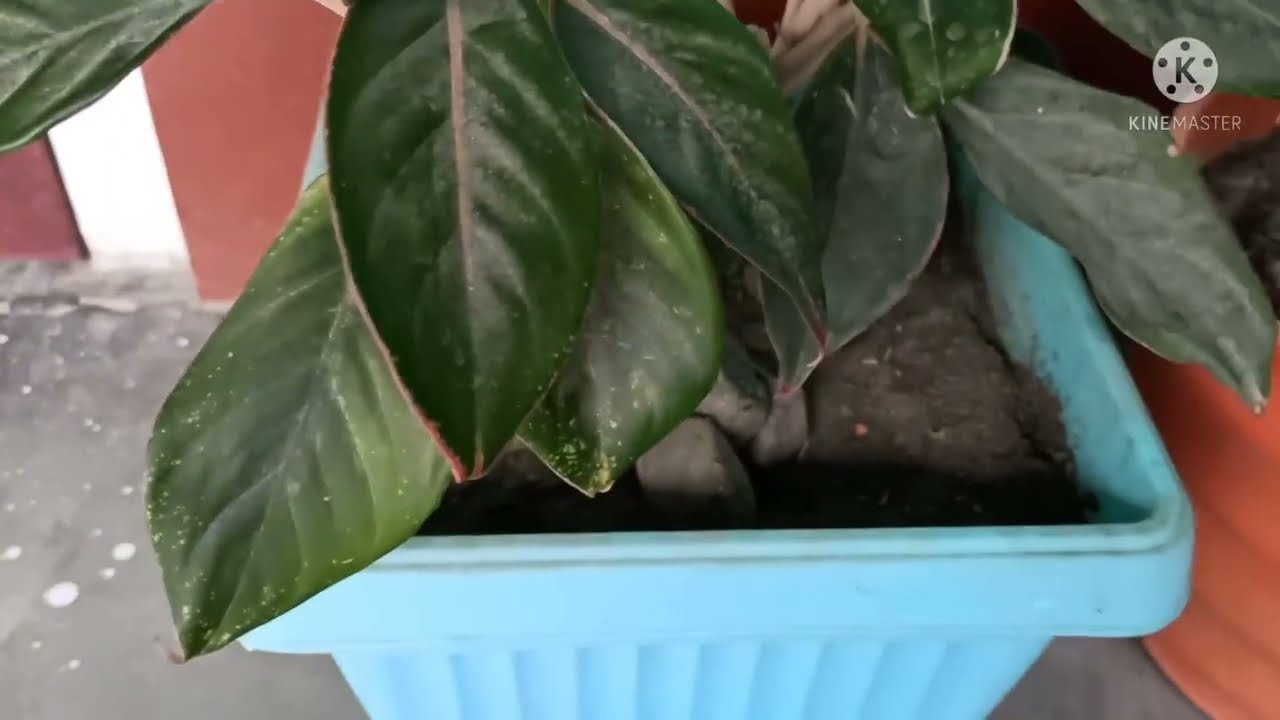The image is a close-up photograph, potentially a still from a video, depicting a potted plant in a light blue, square pot. The plant, which appears to be a rubber plant due to its large, dark green, waxy leaves, is situated in a pot filled with grayish-brown dirt and stabilized with some rocks. The scene likely takes place in a garage or a concrete-covered area, as indicated by the gray floor in the background. The background also features a gray wall behind the planter, with a hint of light shining from behind it. On the far right side of the image, there is an orange object partially visible. Additionally, the image bears a KineMaster watermark in the top right corner, displaying the word "KineMaster" with its corresponding logo of a 'K' inside a white circle surrounded by five dots.